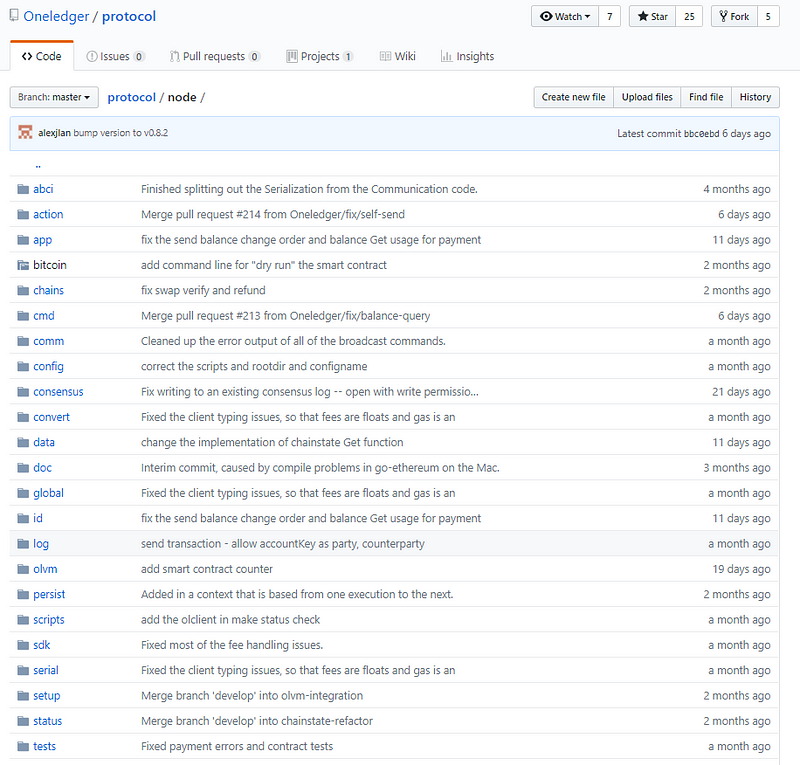This screenshot displays a directory featuring an extensive list of folders. At the top left corner, the heading reads "oneledger/protocol" in blue font. Adjacent to this, on the right-hand side, there are three icons, each accompanied by a counter: a watch icon with the number 7, a star icon with the number 25, and a fork icon with the number 5.

Below this section, there are six distinct tabs. The first tab, "Code," is highlighted with an orange line, indicating it is the active tab. The subsequent tabs are as follows: "Issues" with a count of 0, "Pull requests" showing 0, "Projects" with a count of 1, "Wiki," and "Insights."

Beneath these tabs, on the left side, there is a drop-down box labeled "branch: master." Next to this drop-down, it reads "protocol/node." To the right of this setup, there are four buttons arrayed side-by-side.